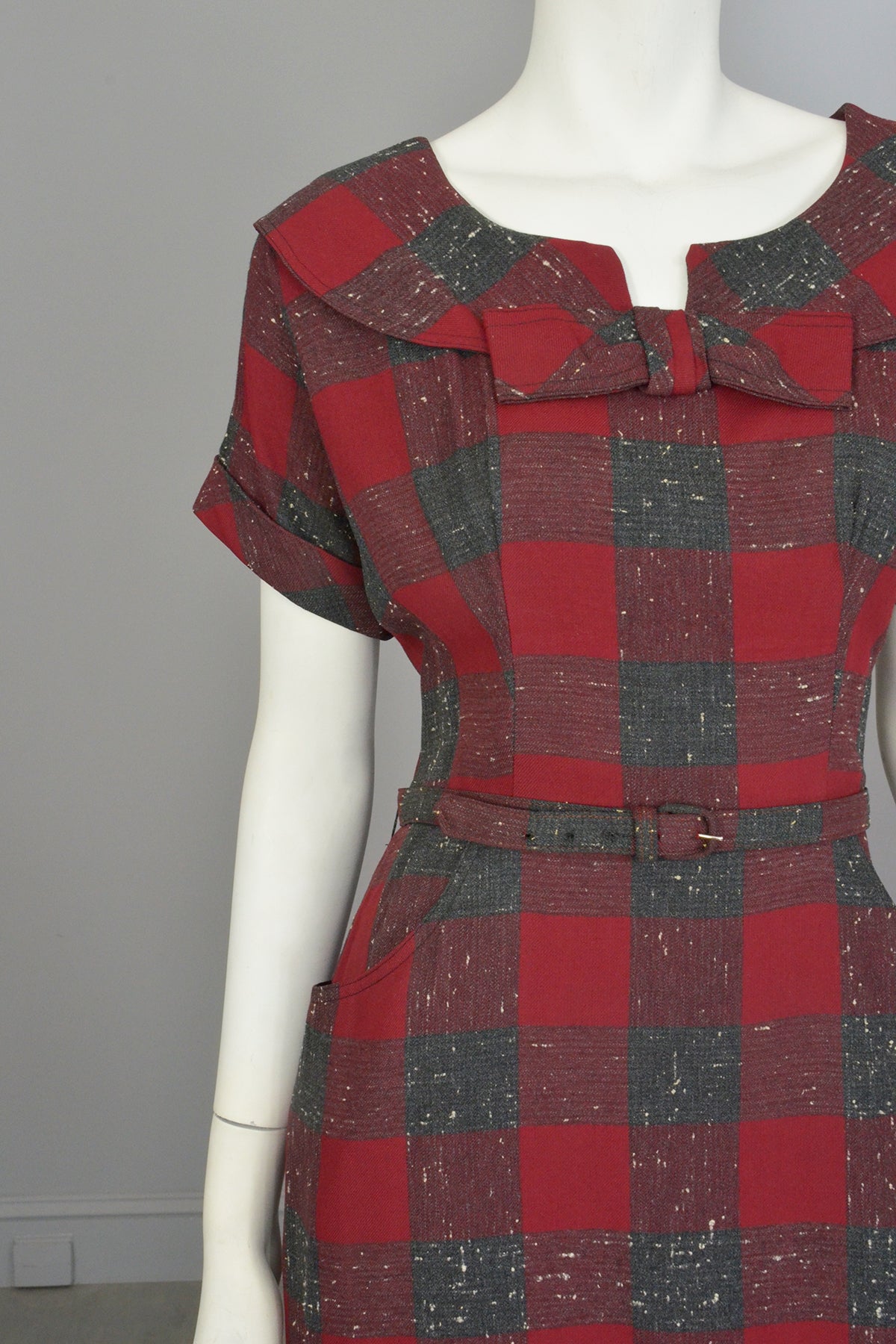In this photograph, a purely white mannequin stands against soft gray walls and a medium gray floor backdrop. The mannequin, cropped at the neck and just below the waist, features an extended right arm, with visible joint details where the hand attaches to the forearm. The mannequin showcases a holiday-themed, one-piece dress that extends below the photographed area, implying it is long. The dress is adorned with a rich dark red and charcoal plaid pattern interspersed with brighter red checks and a slight glittery effect. It features a collar and a prominent bow just below the neckline, short sleeves cuffed at the top, and a matching belt around the waist. Notably, the dress includes pockets, a rare and appreciated detail in women's fashion.